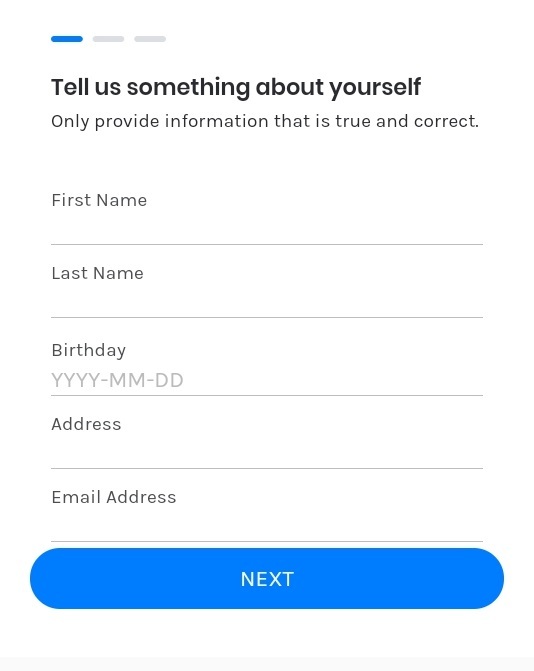The webpage displayed has a clean, white background. In the upper left-hand corner, there are three horizontal dashes: the first one is brightly colored in blue, while the other two are light gray. Immediately below these dashes, bold black text reads, "Tell us something about yourself." Under this heading, there is a line of unbolded black text that says, "Only provide information that is true and correct."

The main section of the page contains a sign-up form. It begins with a label in the upper left corner that reads "First Name," followed by a blank space for input and a long line where users are intended to enter their first name. Directly below, another label reads "Last Name," accompanied by a similar input field and line for the last name.

Next, a "Birthday" label appears, followed by light gray placeholder text indicating the format "yyyy-mm-dd," where users can input their birth date. Below this, the text "Address" is displayed, followed by an empty space for address entry and a bordered input field.

Further down, the form asks for an "Email Address," with an accompanying space and border for email input. 

At the bottom of the form, there is a prominent, bright blue button with a long rectangular shape and rounded corners. Centered on the button, white text reads "Next."